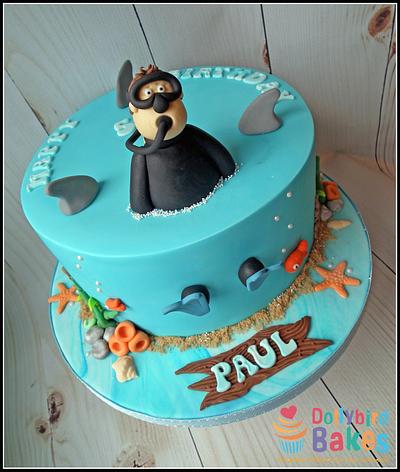This is an image of an intricately designed and festive birthday cake, set against a whitewashed tabletop and back wall. The cake, created by Dolly Bird Bakes as indicated by the logo in the bottom left-hand corner featuring a graphic cupcake, is light blue and themed around a scuba diving adventure gone awry. Adorning the cake is a highly detailed figure of a scuba diver in a black wetsuit, emerging from the cake with a look of pure shock on his wide-eyed expression. Surrounding him are realistic shark fins, reflecting an imminent danger, and the inscription "Happy Birthday, Paul."

The artistry extends to the base of the cake where crumbs have been arranged to resemble sand, and various sea elements like starfish, coral, and seashells made from confectioner's sugar are scattered. Additionally, small pearl-like bubbles are incorporated to enhance the underwater effect, completing the illusion of a lively, underwater scene. Overall, the cake is a vivid, playful, and expertly crafted centerpiece, ideal for a child's birthday celebration.